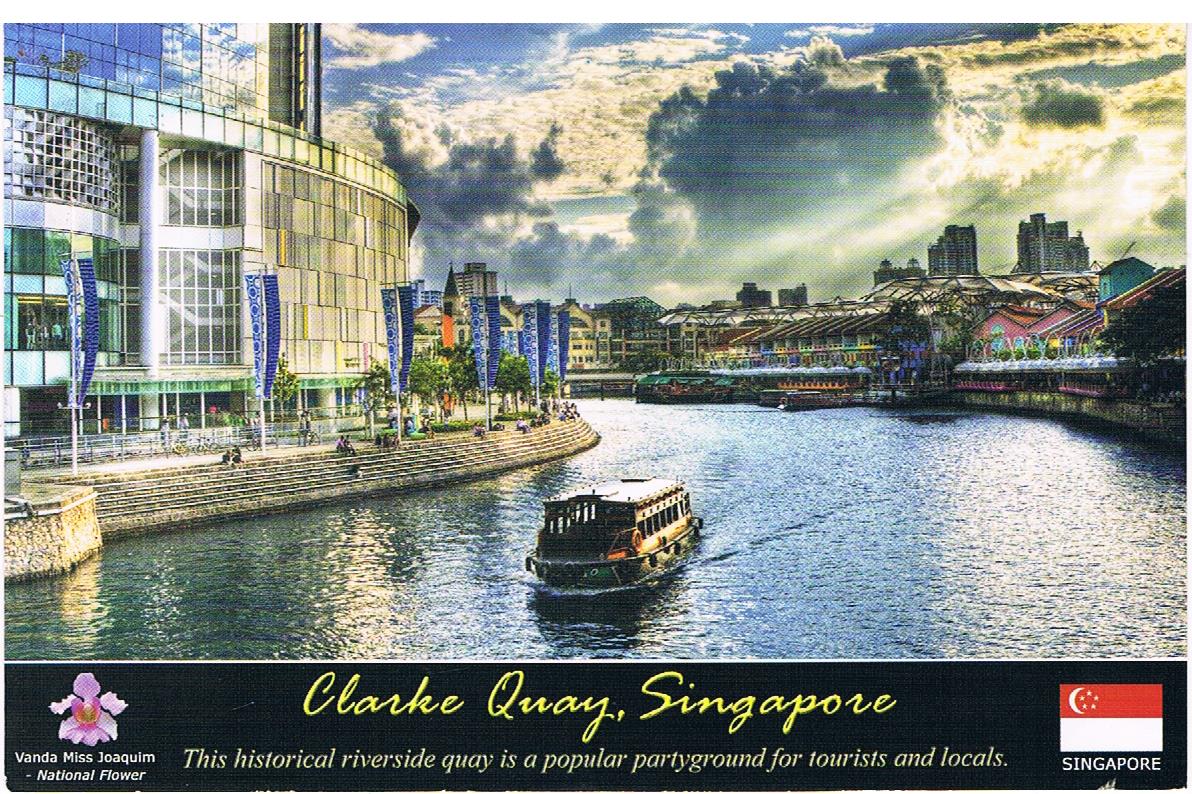In this vibrant, artistic rendering of an outdoor scene on a somewhat cloudy day, we see a river winding like a moat around a large, ornate glass building situated on the left side. This building is enhanced by stone stairs leading down to the water, with blue banners lining the stairway. The center of the river features a riverboat designed for leisure cruising. On the far shore, there are more buildings, some of which are open-air structures with covered tables, adding to a bustling atmosphere. Surrounding these structures are more buildings, including some towering skyscrapers and possibly houses.

Various elements of the image are marked by notable details: at the bottom, a black rectangular banner displays the text "Clark Quay, Singapore" in yellow cursive font. To the left of the text, there is a pink flower—identified as the "Vanda Miss Joaquim, National Flower"—accompanied by a purple emblem. Further to the left, the flag of Singapore is visible, featuring a red background with a white crescent moon and five stars, and the word "Singapore" printed below it. This historical riverside quay, depicted in the image, is celebrated as a popular gathering spot for both tourists and locals.